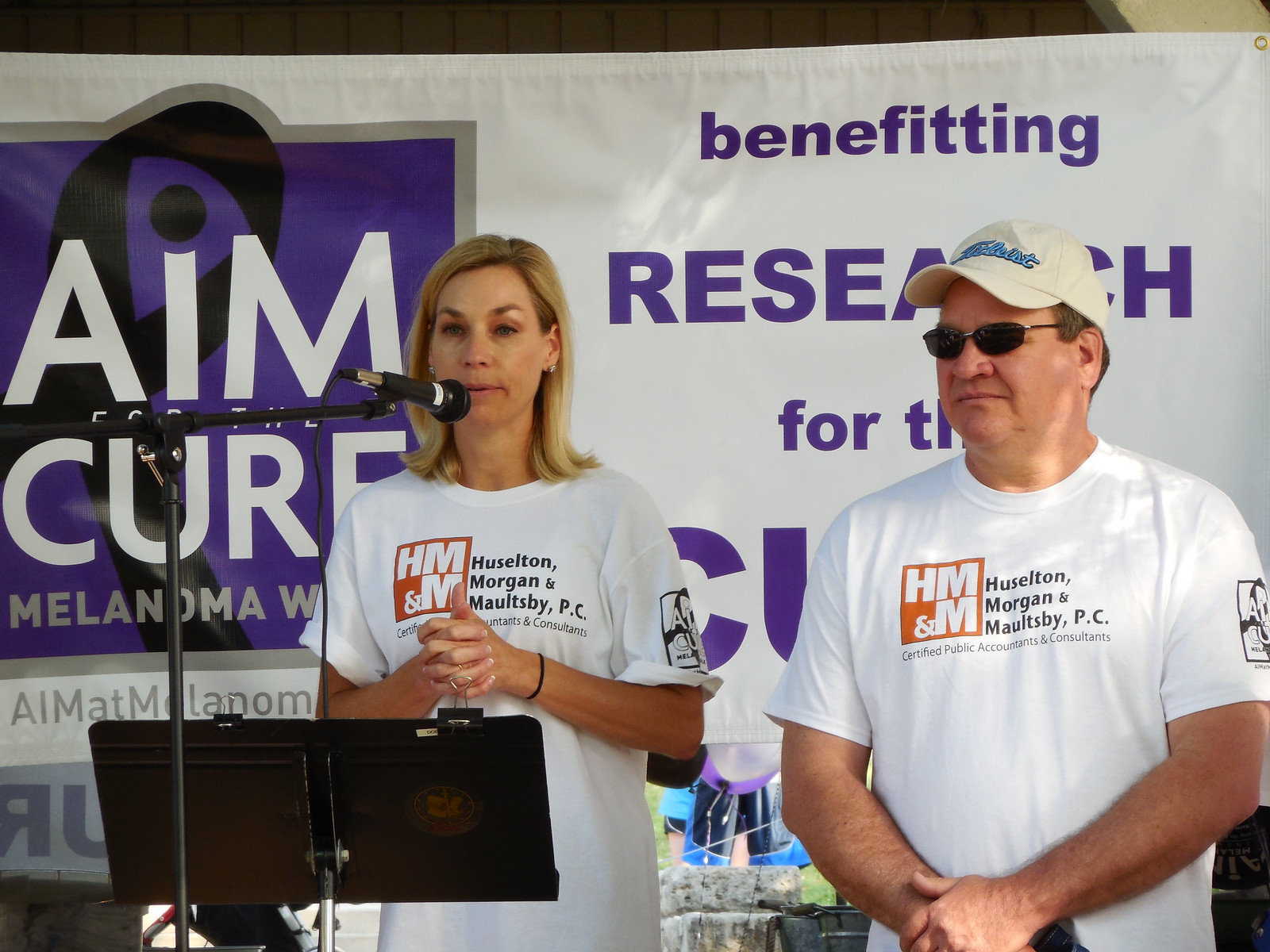In this detailed image, a woman and a man are standing at a podium, giving the impression of being on a stage, perhaps for some charity event. The woman, with blonde hair, is speaking into a microphone attached to a stand, her hands clasped in front of her. She wears a white t-shirt emblazoned with "Hustleton, Morgan, and Maltby PC, Certified Public Accountants and Consultants" along with the logo HMM and M. The man stands adjacent to her, similarly dressed in the same t-shirt, sporting sunglasses and a white baseball cap with red lettering.

Behind them, a large banner predominantly in white and purple is displayed. The upper left corner of the banner features the text "AIM CURE" in white print against a purple background, with "melanoma" written in gray letters beneath it. To the right, partially obscured by the pair, the banner reads "Benefiting Research" in purple lettering, indicating the event's charitable cause. The detailed backdrop and the coordinated attire of the speakers suggest a professional and focused effort toward advancing research for melanoma.